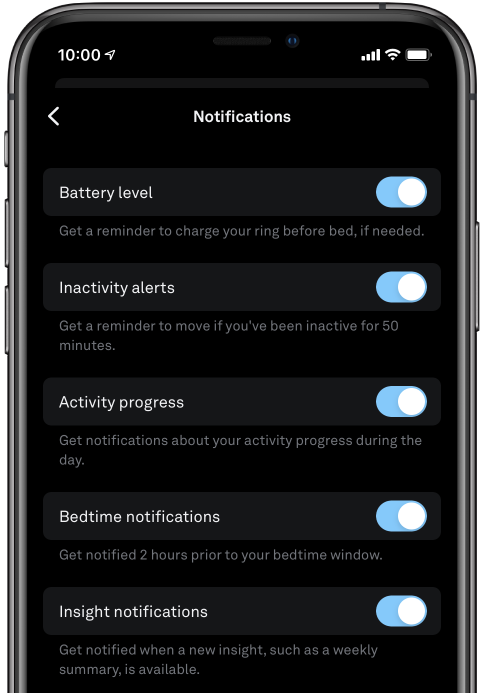**Detailed Caption:**

The image displays a dark-themed interface of a smartphone's notification settings. The background is black with white text, making the elements highly visible. At the top right corner, the battery indicator is shown at full capacity beside a Wi-Fi signal icon. The current time, displayed on the far-left, is 10:00 AM.

The settings options are listed as follows:

1. **Battery Level Notification**: Selected, showing options to receive a reminder to charge the phone or a smart ring before bed if the battery is low.
2. **Activity Alert**: Enabled, providing a reminder to stay active if there has been 50 minutes of inactivity.
3. **Activity Progress**: Turned on, sending updates about daily activity milestones.
4. **Bedtime Notifications**: Activated, giving a notification two hours before the user's set bedtime.
5. **Insight Notifications**: Enabled, offering insights such as weekly summaries when available.

Each notification setting has a slider button colored light blue with a white dot aligned to the extreme right, indicating that it is turned on.

The interface also includes an image of a phone outline on the right, which illustrates volume control buttons on the left side and a power button on the right side. An additional feature shown is a button to silence all notifications entirely.